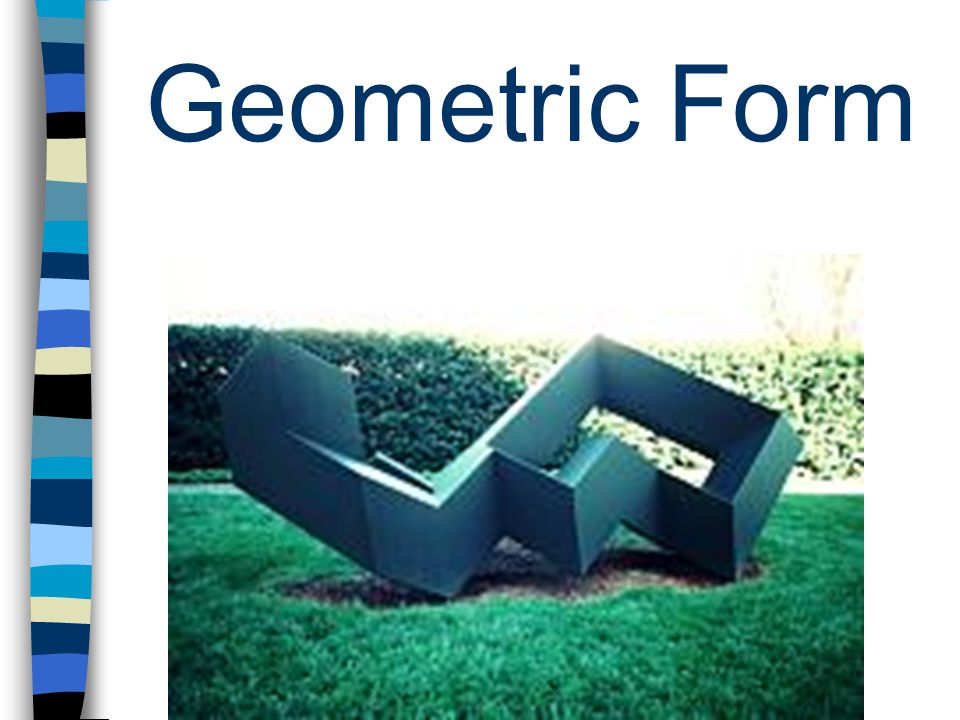The image presents a composition titled "Geometric Form," which is prominently displayed in large blue lettering at the top. On the far left, a digitally-created column with a narrow top is set against a white background. This column features stripes in various shades of blue, including teal, greenish-blue, dark blue, light blue, interspersed with black, off-white, and beige, and extends vertically to the bottom of the image. Moving towards the center, the image transitions to an outdoor scene with a vivid green lawn and a meticulously trimmed hedge. Sitting at the center of this grassy area is a dark green metal sculpture characterized by its complex and curvilinear shapes. The sculpture exhibits many square-like curves, forming an abstract, multifaceted geometric structure. The overall setting resembles a slide from a presentation, possibly created using software like PowerPoint.